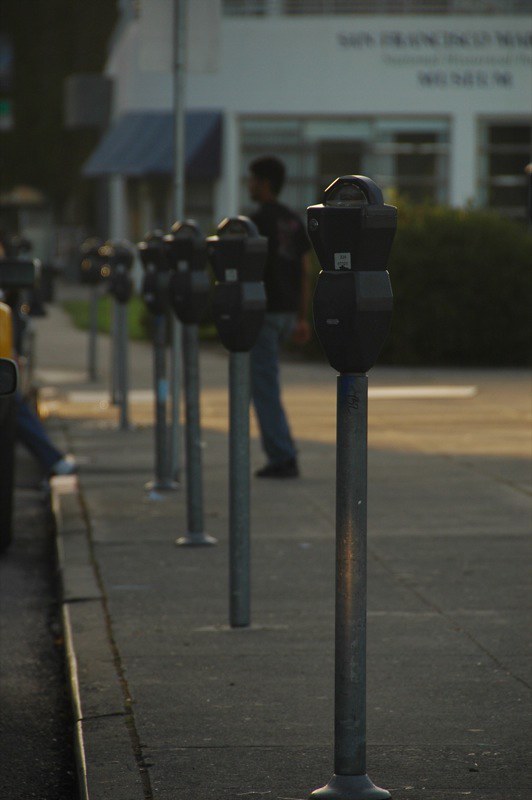This somewhat low-light color photograph captures a city sidewalk scene featuring a row of six parking meters attached to silver poles with black tops, likely coin-operated, aligned along the curb. The meters stretch into the distance, fading into the background. On the sidewalk, a pedestrian in a black shirt and blue jeans walks away from the viewer, partially cloaked in shadow, with soft light falling across the ground in front of him suggesting the setting sun. Behind the pedestrian is a white concrete building with blue awnings, decorated with shrubbery and hedges in front, and an indistinct string of letters on its facade indicating some sort of establishment, possibly a post office. The scene includes a hint of vehicles parked along the curb, though they remain largely indiscernible, contributing to the overall muted, shadowed ambiance.